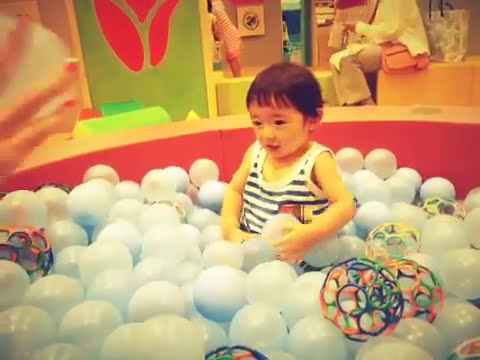This image features a small Asian toddler joyfully playing in a vibrant ball pit. The child has short black hair with bangs and is wearing a sleeveless, horizontally striped tank top in black and white. They are seated amidst predominantly light bluish-white plastic balls that fill the lower half of the image. The ball pit itself has a red rim and contains a few multicolored geodesic spheres scattered among the other balls. In the background, the walls are painted light green and decorated with a red tulip and hints of orange and pink. Seated behind the child is an older woman, visible from the waist down, dressed in a light-colored sweater and tan pants, with a pink purse at her side. Additionally, the seating area behind her includes colored rectangular seats in shades of yellow and light green. Another child, dressed in a striped dress, is also seen in the background, engaged in an activity within this lively play area for children.